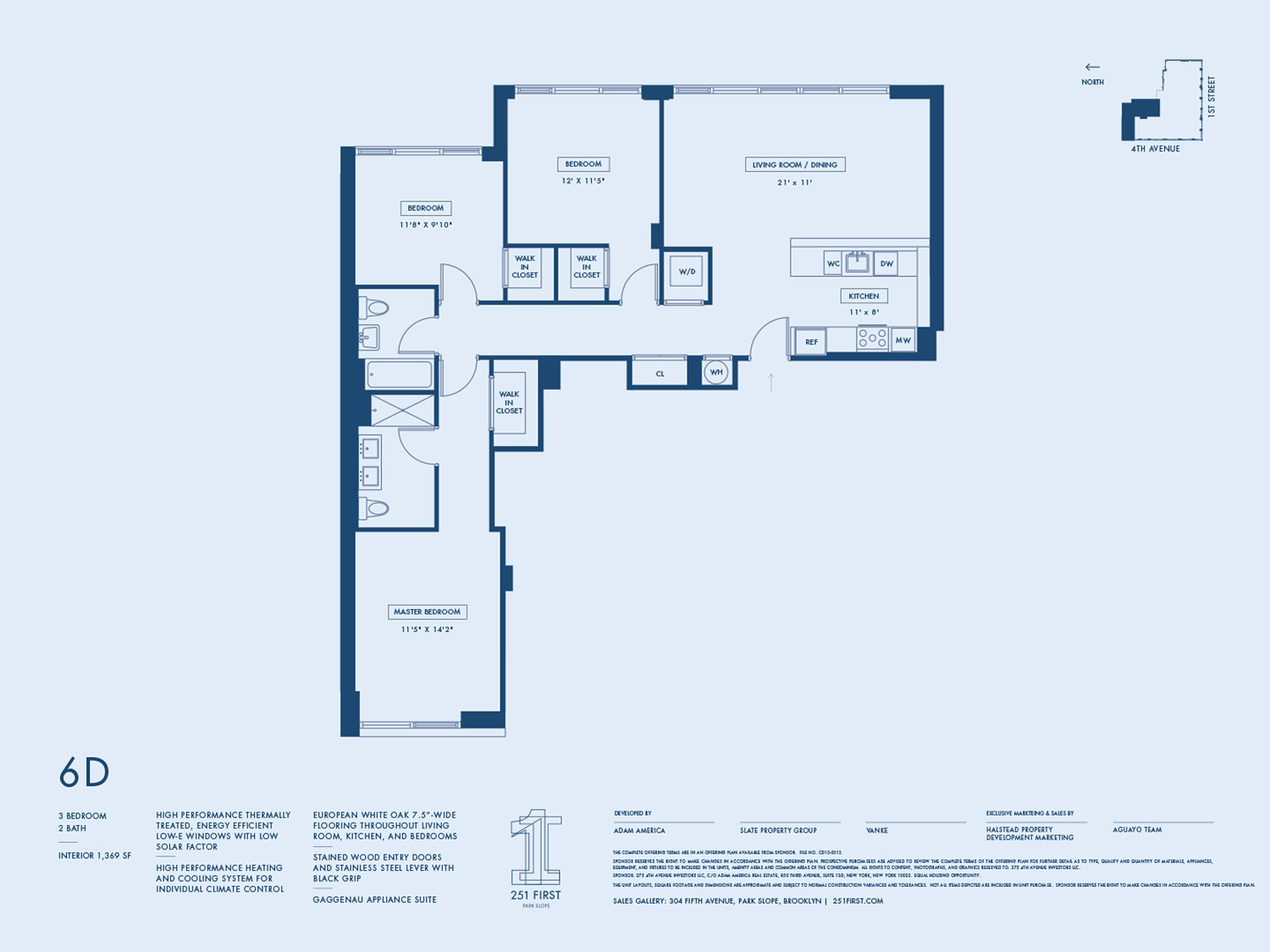This image displays a detailed floor plan of an apartment with a light blue background. In the bottom left corner, the label "6D" is prominently displayed, and although the text is small, it indicates that the layout is for a three-bedroom, two-bathroom apartment. Each room is clearly marked, albeit with tiny text. 

The master bedroom is labeled, along with other essential areas such as the living room, kitchen, restroom, walk-in closet, and a washer/dryer area. The entrance is indicated by an arrow pointing towards a symbol that resembles a door swung open. Upon entering, you walk into the living room. Turning left from there leads to a restroom and a bedroom. Taking another left turn from that path directs you to the master bedroom. 

The exact square footage is difficult to discern due to the small text, but it appears to be around 1,200 square feet.